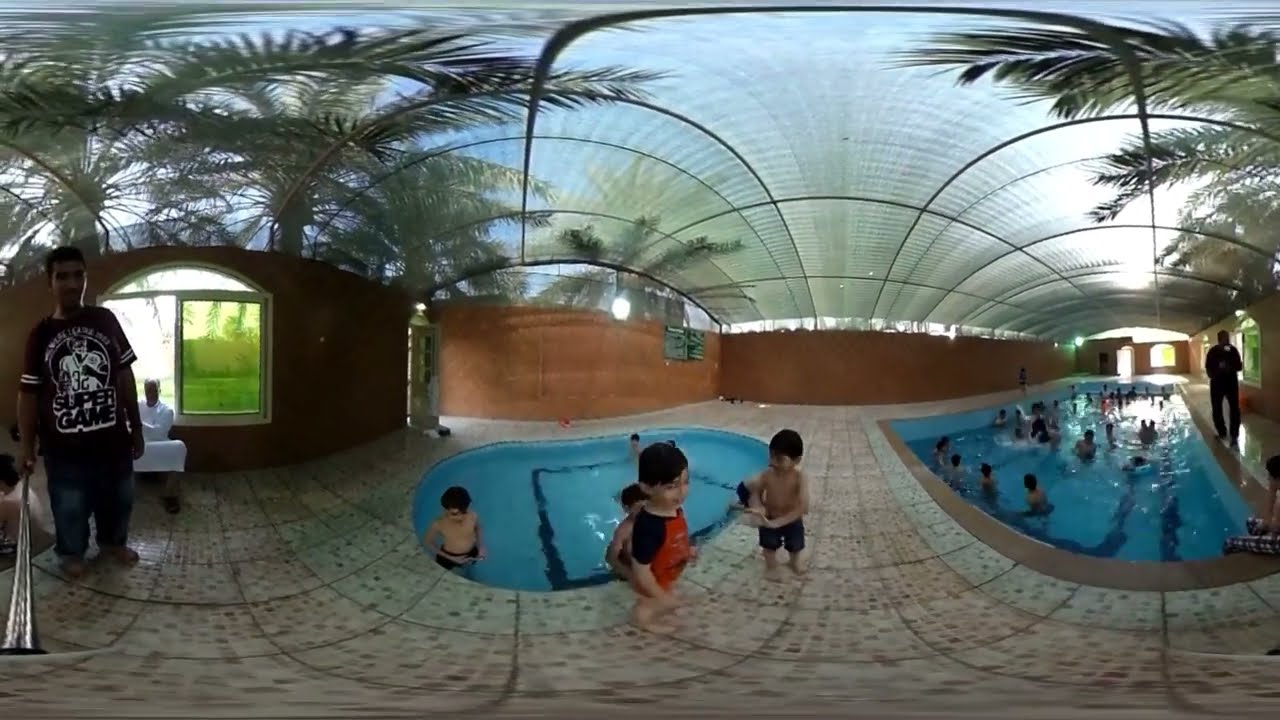In this panoramic photograph, the viewer looks down on a bustling swimming pool brimming with people, their swim trunks vividly contrasting the light blue water. The pool, which curves from the bottom left corner to the upper right corner due to the lens distortion, features dark blue lines at its bottom. Surrounding the pool on the left and right sides are walkways made of light brown panels held together by brown mortar. Behind these walkways, wooden-colored walls encircle the pool, adorned with arches outlined in black lines that reveal lighter gray lines beneath. Centered above, a brilliant white light from the sun shines through. On the right side of the pool area, tall palm trees extend upwards, their green leaves almost reaching the top of the image. 

Additional details include multiple bodies of water situated far left and far right of the main pool. To the left, a round-shaped pool is visible, beside which stands a man in a black shirt with circular patterns on the sleeves and black pants. On the right, a young man in knee-length shorts stands by another body of water. The pool area appears to be outdoors with buildings visible in the distance and a net covering partially shading the scene. The color palette in the image features a mix of blues, greens, browns, and other vibrant hues. The setting suggests a public pool, alive with daytime activity under the approximately clear sky.